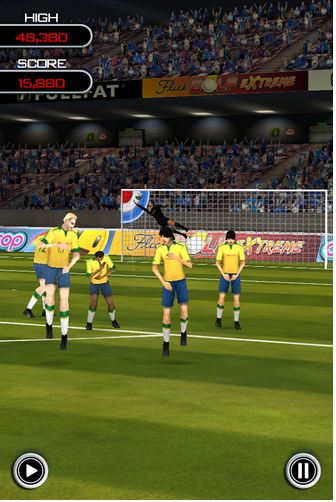This is a detailed screenshot from a video game simulating a soccer match. The scene captures a vibrant stadium with rows of colored dots representing the audience. The playing field, alternating between light and dark green, features a white net in the back where a player in black is leaping towards the upper left corner to intercept a soccer ball. At the forefront, five players wearing yellow shirts, blue shorts, and white stockings with green bands are seen in dynamic poses, seemingly suspended in mid-air. 

In the upper left corner of the screen, the text "HIGH" appears in white, followed by red numbers displaying a high score of 48,380. Below that, the word "SCORE" is written in white, accompanied by an orange figure of 15,880. On the bottom left corner, a circular play button with a white triangle is seen, whereas the bottom right corner houses a pause button represented by a circle with two vertical bars. This very detailed scene portrays an animated and immersive soccer game environment.